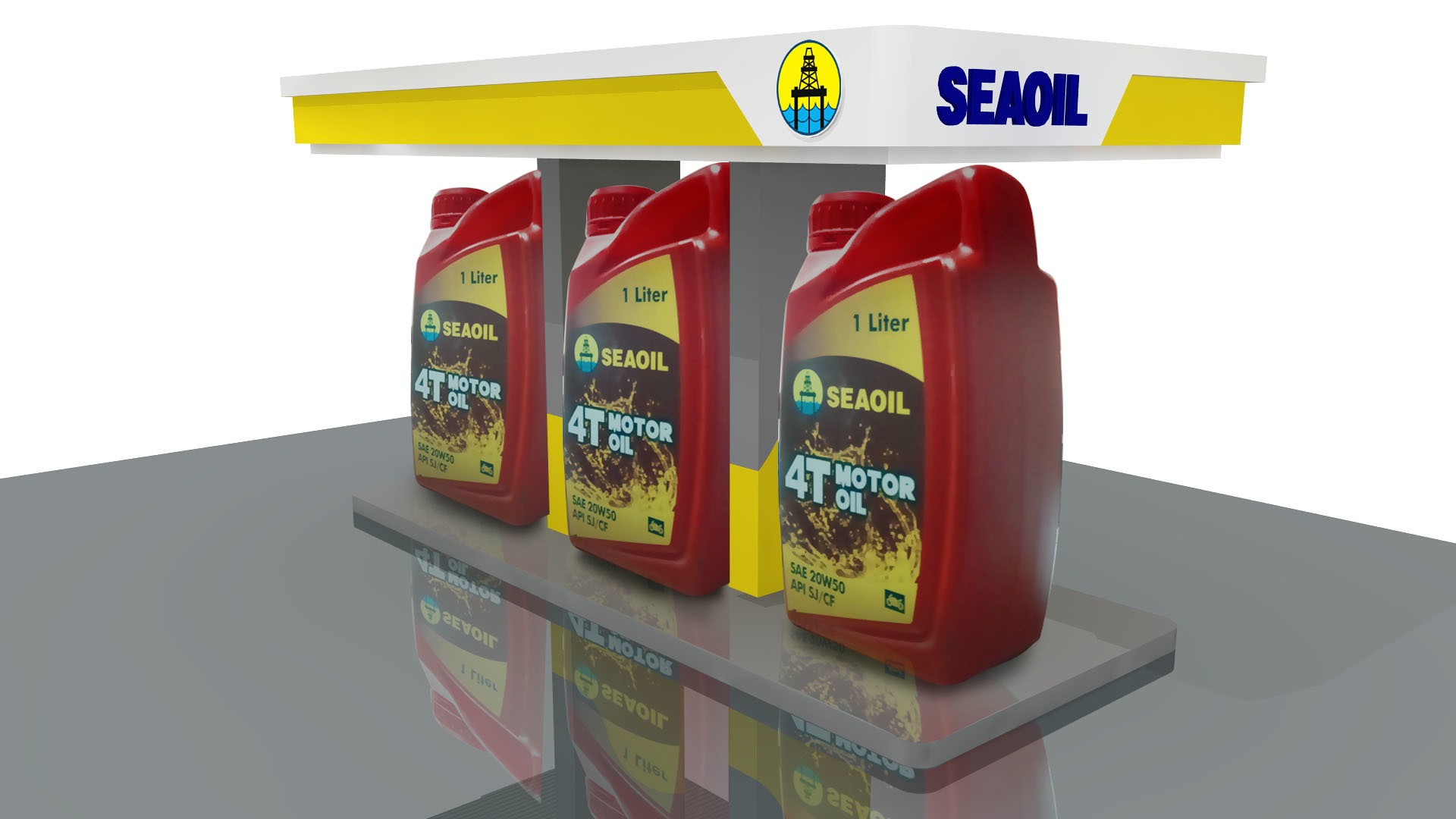The image depicts a digital rendering of three red 1-liter motor oil containers, each adorned with yellow labels featuring the black text "C-Oil" and "4T motor oil" in white. The containers are centrally positioned on a shiny, gray, reflective surface that resembles a clean, hard table. They are arranged side by side, beneath a digitally drawn structure resembling a gas station podium with a white and yellow roof. At the top of this podium, "C-Oil" is displayed in blue letters, accompanied by a logo with a yellow background and a blue 'C' featuring an oil rig. The background of the image is a solid white, providing a stark contrast to the vibrant colors of the motor oil containers and the podium setup. The overall arrangement and the reflective surface suggest an indoor setting, possibly in a showroom or an auto body shop.